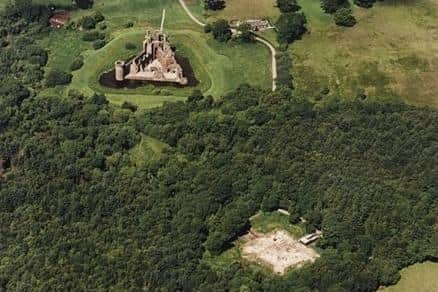The aerial image showcases an ancient, triangular-shaped stone castle, possibly medieval, at the top center of a verdant field. The castle is surrounded by a thick, dark green forest, likely consisting of evergreen trees with dense canopies. To the bottom right of the image, there is a noticeable beige, empty section of land, which contrasts with the lush, green grassy areas around it. A path leads from this barren patch towards the castle. Additionally, the castle appears to be encircled by a moat and hills, enhancing its fortified appearance. The surrounding forest is expansive and dense, except for a distinct clearing where it seems a structure once stood but has since been demolished, leaving a grey residue. This high-resolution, possibly computer-generated or drone-captured image, vividly captures a scene reminiscent of ancient architectural styles and landscapes.